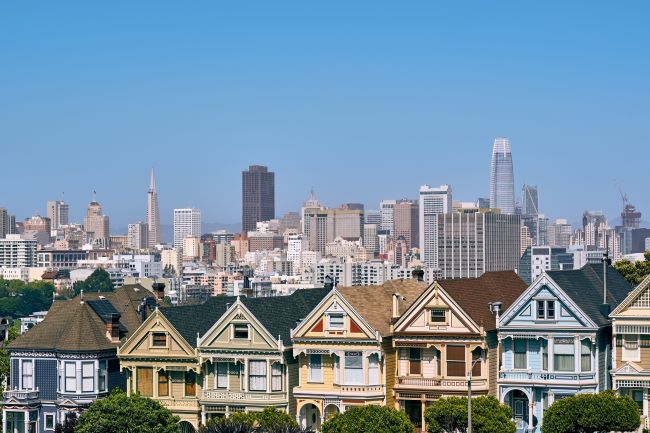A vibrant, outdoor aerial photograph captures a picturesque cityscape. In the foreground, there is a row of six charming, multi-story townhouses, reminiscent of San Francisco's iconic architecture, featuring rich, varied facades in hues of green, blue, cream, and tan. Each home has two main levels topped with an attic, showcasing numerous windows and intricate details. A seventh house appears partially cut off on the right edge of the image. In front of these elegant homes, the tops of lush, verdant trees are visible, their green leaves providing a natural contrast to the urban scene. The midground transitions to a bustling downtown area filled with soaring skyscrapers in shades of white, cream, silver, and black. The entire scene is set against a brilliant, cloudless blue sky, lending a bright, vibrant feel to this cityscape blending residential charm with metropolitan grandeur.